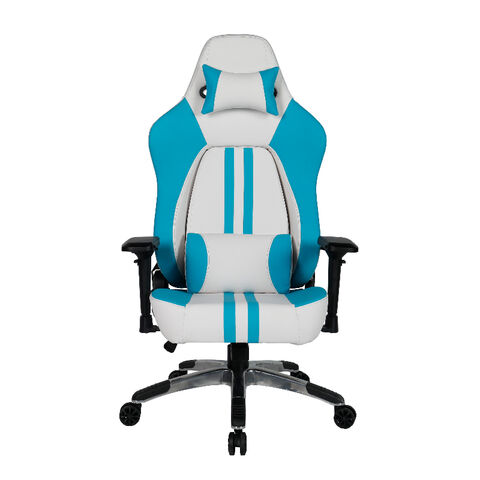The image displays a gaming chair set against a plain white background, emphasizing its sleek and ergonomic design. The chair features a striking color scheme of blue and white for the body, complemented by black armrests, a black base, and black rollers. It boasts a high backrest with two prominent turquoise racing stripes running vertically down both the back and seat areas, providing a dynamic and sporty look. The edges of the backrest and seat are accented with blue turquoise, enhancing the chair's modern aesthetic. Attached to the chair are two cushions: a headrest pillow and a lumbar support pillow, both in white with blue turquoise edges, ensuring added comfort and proper neck and spine support. The chair is equipped with five legs and adjustable seat features, making it ideal for gaming or extended computer use. The front view clearly showcases these details, emphasizing its functionality and style.